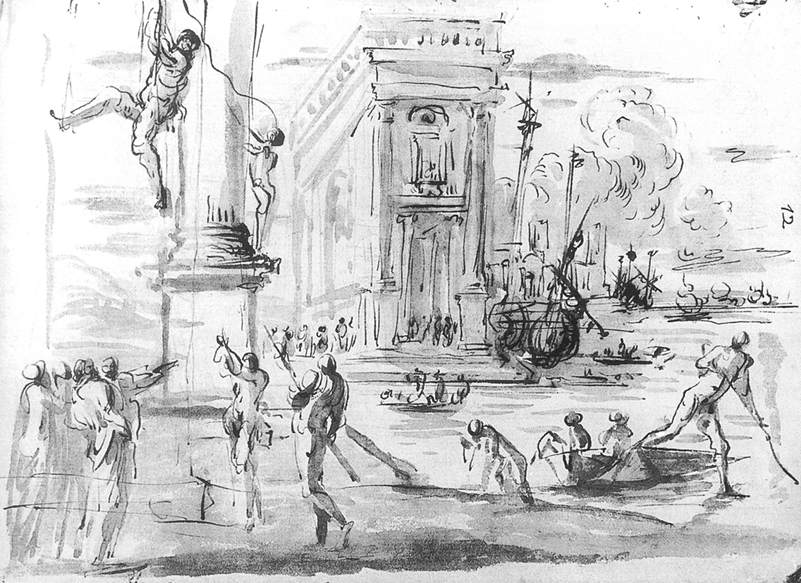This black and white drawing is centered around a large, arched building with grand columns flanking a main door, above which an inset statue is perched. The building, reminiscent of a town hall, extends towards the left background and stands near a river. Clouds fill the sky, rendered in varying shades of gray. 

On the left, several men are climbing a tall flagpole using ropes, while below, a group of white-robed figures points guns skyward. Further left, a small boat with two seated individuals floats on the river. Across from the main building, on the far side of the river, stands another tall structure, possibly another building.

In the foreground, there are naked figures brandishing sticks or spears, contrasting with the robed figures near the flagpole. On the far right, a lone individual is actively pulling on a rope. A secondary boat is positioned mid-river, adding to the dynamic scene. The setting is entirely in shades of gray, black, and white, with the only discernible text being a sideways number "12" inscribed on the right side, though it might be a vague scribble. This intricate and detailed illustration combines elements of surrealism and historical style, offering a vivid and chaotic tableau.